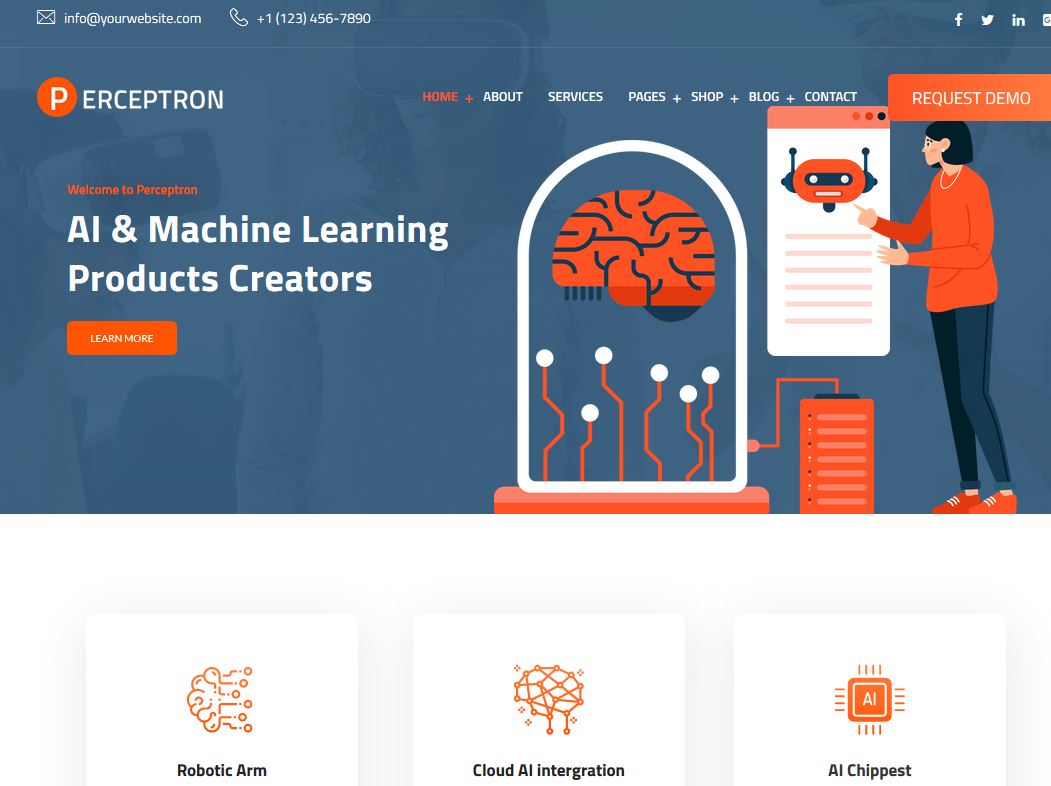The screenshot depicts the homepage of a website called Perceptron. The website's title is prominently displayed in the top left corner, featuring a stylized 'P' within an orange circle, followed by the text "Perceptron" spelled out (P-E-R-C-E-P-T-R-O-N). The website's color scheme is composed of shades of blue, primarily leaning towards a grayish blue, complemented by vibrant orange accents and white backgrounds.

The page's art style is minimalistic, utilizing flat colors and simple shading. Dominating the upper portion of the homepage is a welcoming banner that reads "Welcome to Perceptron" with a subtitle stating "AI and Machine Learning Product Creators." Below this text is an orange button labeled "Learn More." 

On the right side of the banner, a graphic illustration showcases a brain encased in a glass jar and connected to various mechanical devices. This visual is also minimalistic and pairs well with the adjacent image of a young woman pointing towards a poster or depiction of a robot.

The navigation bar at the top includes several sections such as Home, About, Services, Pages, Shop, Blog, and Contact. The labels Home, Pages, Shop, Blog, and Contact each have a plus sign, indicating expandable submenus. Currently, the Home section is selected.

Towards the bottom of the screenshot, three selectable categories are displayed: Robotic Arm, Cloud AI Integration, and AI Chip Test, each possibly leading to more detailed content within the site.